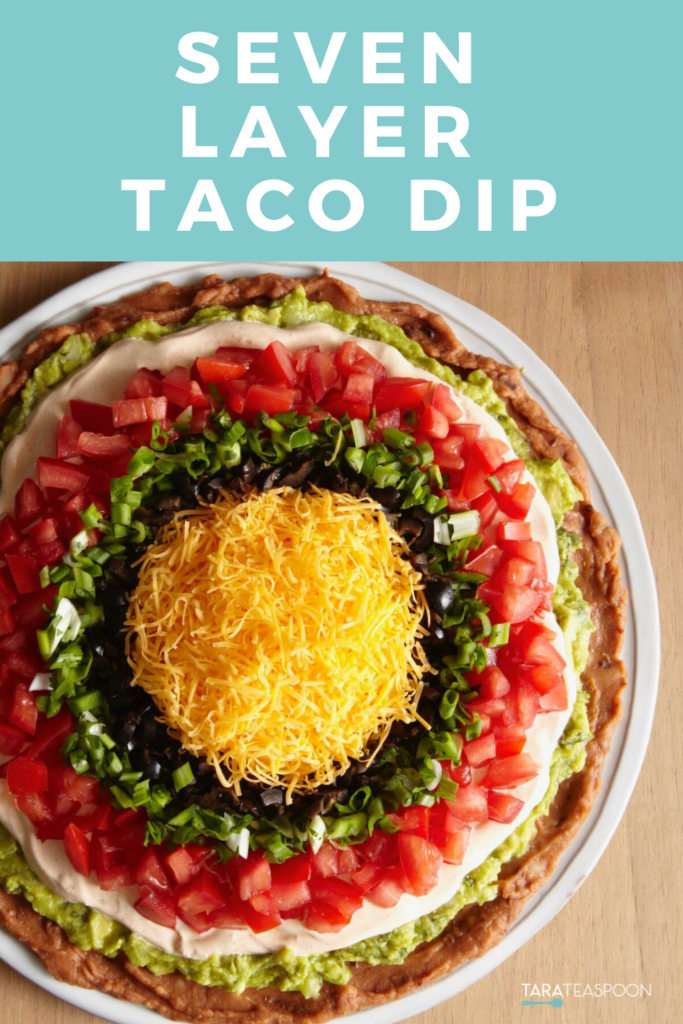This detailed poster features a professionally prepared, stock image of a perfectly circular seven-layer taco dip. At the top, a light pale blue box stretches across the entire width of the poster, adorned with white block lettering that prominently reads "Seven Layer Taco Dip." Below this header, the realistic image of the dip is displayed, revealing each meticulously organized layer. Starting from the bottom, the layers include beans, creamy guacamole, white sour cream, diced red tomatoes, green onions, chopped black olives, and a topping of yellow fiesta cheese. The dish is presented neatly on a white plate that rests on a wood grain table, evoking a homely, recipe-book feel. In the bottom right corner of the poster, the logo "Terra Teaspoon" is visible, featuring a small blue teaspoon icon beneath the text. The entire presentation suggests a high level of care and professionalism, making the dip look both delicious and inviting.